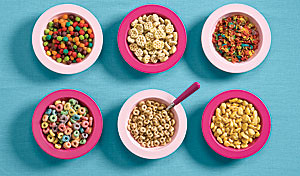The image depicts six bowls of cereal arranged in a neat 3x2 grid on a light blue or turquoise surface. The bowls alternate in color: the top row features a light pink bowl, a dark pink bowl, and another light pink bowl, while the bottom row reverses the pattern with dark pink, light pink, and dark pink bowls. The image is taken from a top-down perspective, allowing a clear view of the cereal types. 

From left to right, the cereals in the top row are:
1. Colorful puffs, resembling Trix.
2. Honeycomb-shaped cereal pieces.
3. Brightly colored pebbles akin to Fruity Pebbles. 

In the bottom row, from left to right, the cereals are:
1. Colorful loops, likely Froot Loops.
2. Brown Cheerios, with a spoon featuring a dark pink handle dipped inside.
3. Yellow, puffed cereal similar to Corn Pops.

The bowls cast shadows towards the bottom left, indicating the light source is coming from the top right.